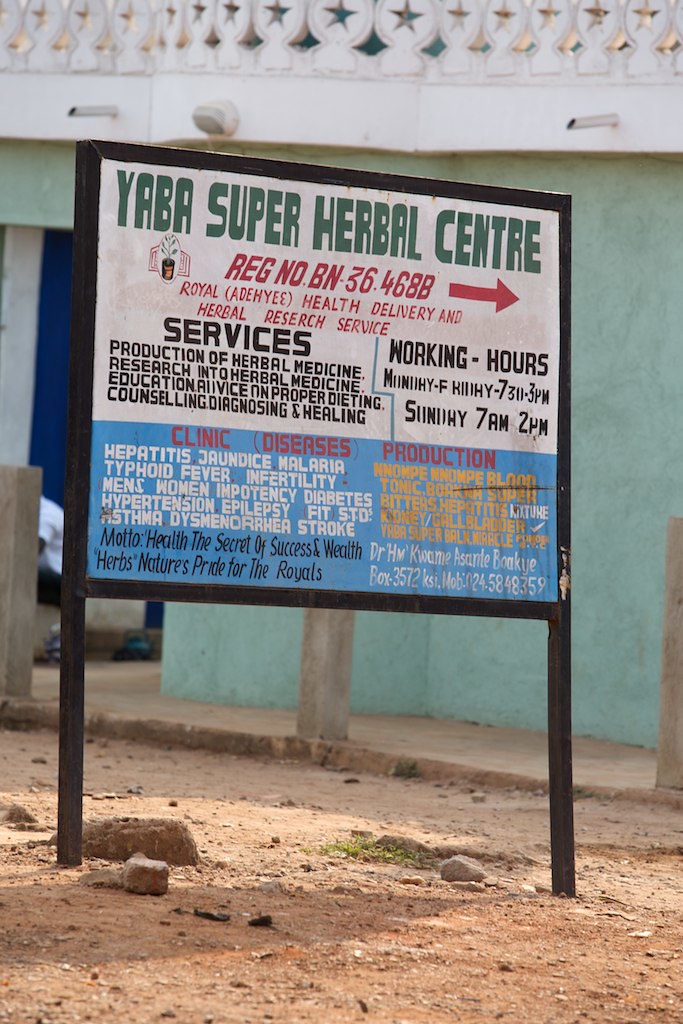The image features a weathered sign standing on two posts planted in a dirt area scattered with rocks. Sparse plant life, including one noticeable weed, is visible around the base. Behind the sign, a light blue building with a few wooden posts adds context to the rural setting.

At the top of the sign, large green letters proudly announce "YABA Super Herbal Center," with additional details including "Region Number BN36468B" and the name "Royal Adehiye" in parentheses. Clearly, this establishment provides a variety of services, explicitly noting "Health Delivery and Herbal Research Services." The list of services offered includes the production and research of herbal medicine, education, advice on proper dieting, counseling, diagnosis, and healing.

Specific hours of operation are provided, varying by day: Monday to Friday from 7:30 AM to 3:00 PM, and Sunday from 7:00 AM to 2:00 PM. The sign also highlights their focus on treating numerous ailments such as Hepatitis, Malaria, Typhoid Fever, Diabetes, Hypertension, Epilepsy, STD, Asthma, and Stroke, among others. 

The bottom part of the sign features a blue section with more information in black, white, and yellow lettering. It conveys their motto, "Health, The Secret of Success and Wealth," and champions the use of herbs with the slogan, "Herbs, Nature's Pride for the Royals." Contact details for Dr. HM Kwame Asante-Bakai are also provided, reinforcing the African roots of this herbal center.